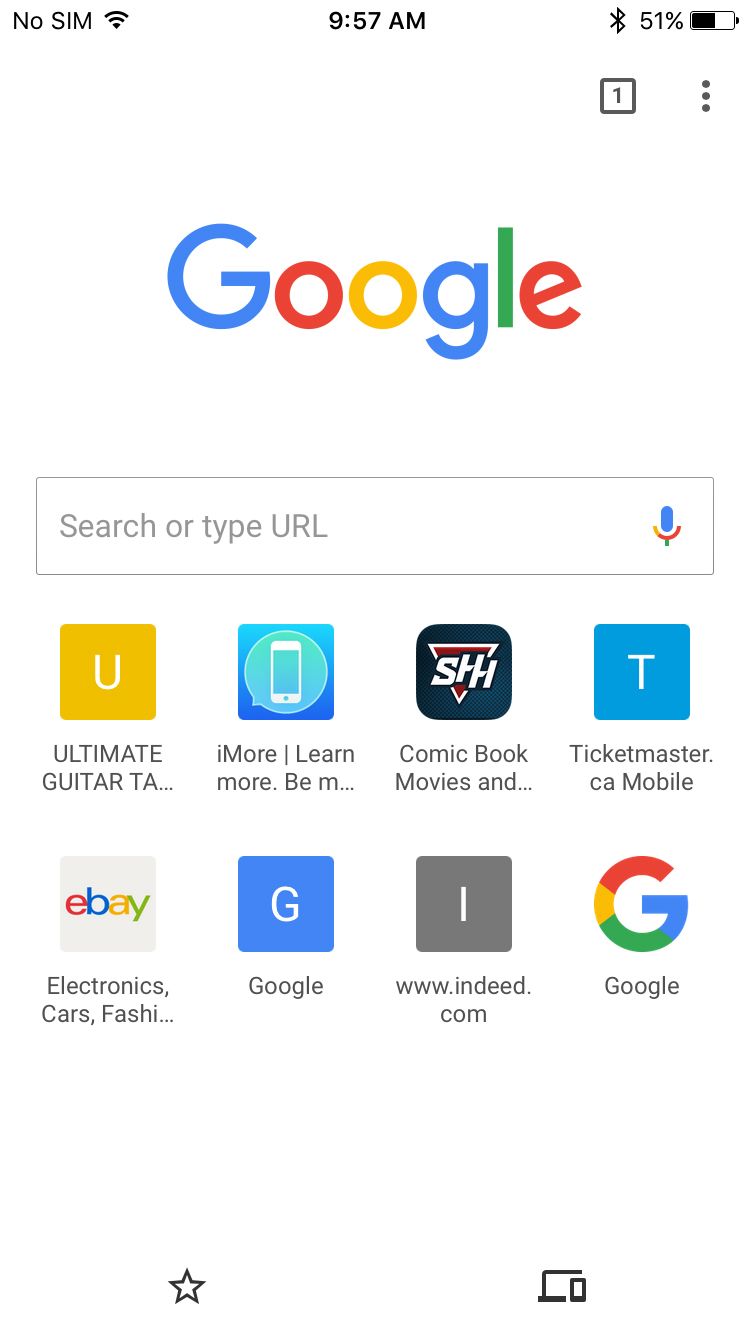This image captures a screenshot of the Google mobile app interface. At the top left, it indicates that there is no SIM card, and the current time is 9:57 AM with a battery level of 51%. There's also a notification icon suggesting that there is one unread message. 

The Google logo is prominently displayed below this, with the search box located directly underneath. This search box allows users to input a search query or type a URL. Below the search box, there are eight frequently visited or favorited options displayed as icons. These icons represent:

1. Ultimate Guitar Tabs 
2. iMore (a resource for learning various things)
3. SHH app (likely a comic book-related resource)
4. Comic Book Movies (another comic book-related resource)
5. Ticketmaster Canada mobile app
6. eBay
7. Google
8. Indeed.com

These options allow for quick access to these sites. There is also a star option, which likely serves as a bookmarking feature, and an option to send search information to another device, such as a laptop or tablet. Another notable feature is the microphone icon, which allows users to conduct voice searches instead of typing. 

Overall, this screenshot provides a detailed view of the Google search experience on a mobile device, reflecting user preferences and frequently accessed sites for convenience.